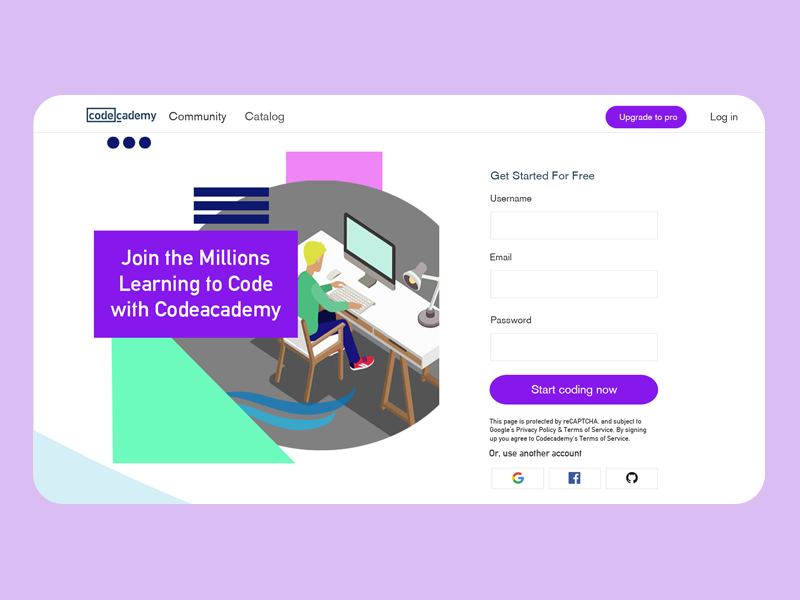This is an image of a website screenshot, featuring a predominantly purple background that gradually transitions from a darker shade at the top to a lighter shade towards the bottom. Centrally positioned is a white, horizontally-oriented rectangle with rounded edges.

At the top left of this white area, bold black letters spell out "Code Academy." To the right of "Code Academy," there are the words "Community" and "Catalog," also in black letters. Adjacent to these, on the far right, is a purple button with the text "Upgrade to Pro" in a lighter purple shade. Further right, the word "Login" appears in black.

Below this header, on the left side, there are three black dots arranged vertically. Directly beneath these dots is an image of a person with brown skin and blonde hair, seated at a computer desk, hands poised over a keyboard. A lamp illuminates the person, casting light in their direction.

Behind the person, there is a blue rectangle with the text "Join the Millions Learning to Code with Code Academy" in white. To the right, against the white background, is the black text "Get Started for Free." 

Further down, a labeled input field "Username" appears in black text with an empty box outlined in gray below it. This is followed by another labeled input field "Email" with an empty, gray-outlined box. Just beneath that, the label "Password" appears, accompanied by another gray-outlined rectangle for input.

Continuing downwards, there is a purple oval button with the words "Start Coding Now" in a lighter purple. At the very bottom, a black text note states, "This page is protected by CAPTCHA and subject to Google's privacy policy and terms of service. By signing up, you agree to Code Academy's terms of service."

Below this note, the text "Or Use Another Account" is displayed in black, followed by three buttons. The first button features the Google symbol, the second has a Facebook logo on a white button, and the third button displays a symbol resembling a 90% closed circle.